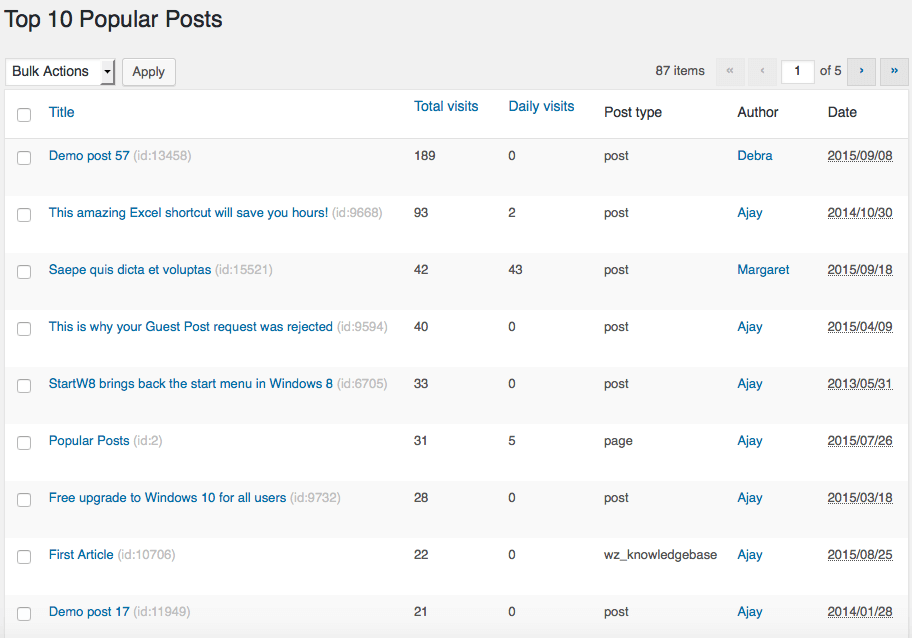The image depicted is a screenshot of a computer screen displaying a content management interface for blog posts. The interface features a gray header at the top. In the top left corner, there are several filter options labeled "Top 10 posts," "Popular posts," followed by "Bulk actions" and an "Apply" button.

Below the header, the interface is organized into a table with columns labeled "Title," "Total Visits," "Daily Visits," "Post Type," "Author," and "Date." On the left side, there is a vertical list of blog post titles, starting with "Demo Post 57," followed by "This Amazing Excel Shortcut Will Save You Hours," "This is Why Your Guest Post Request Was Rejected," "Start WB Brings Back the Start Menu in Windows 8," "Popular Posts," "Free Upgrade to Windows 10 for All Users," "First Article," and "Demo Post 17."

Each blog post entry is accompanied by metrics on total visits, daily visits, post type, author, and date, arranged in columns to the right of the post titles. The text for post titles, daily visits, total visits, and author names is highlighted in blue, while the remaining text is black.

In the top right corner of the interface, it indicates that there are 87 items, with the current view displaying page 1 of 5.